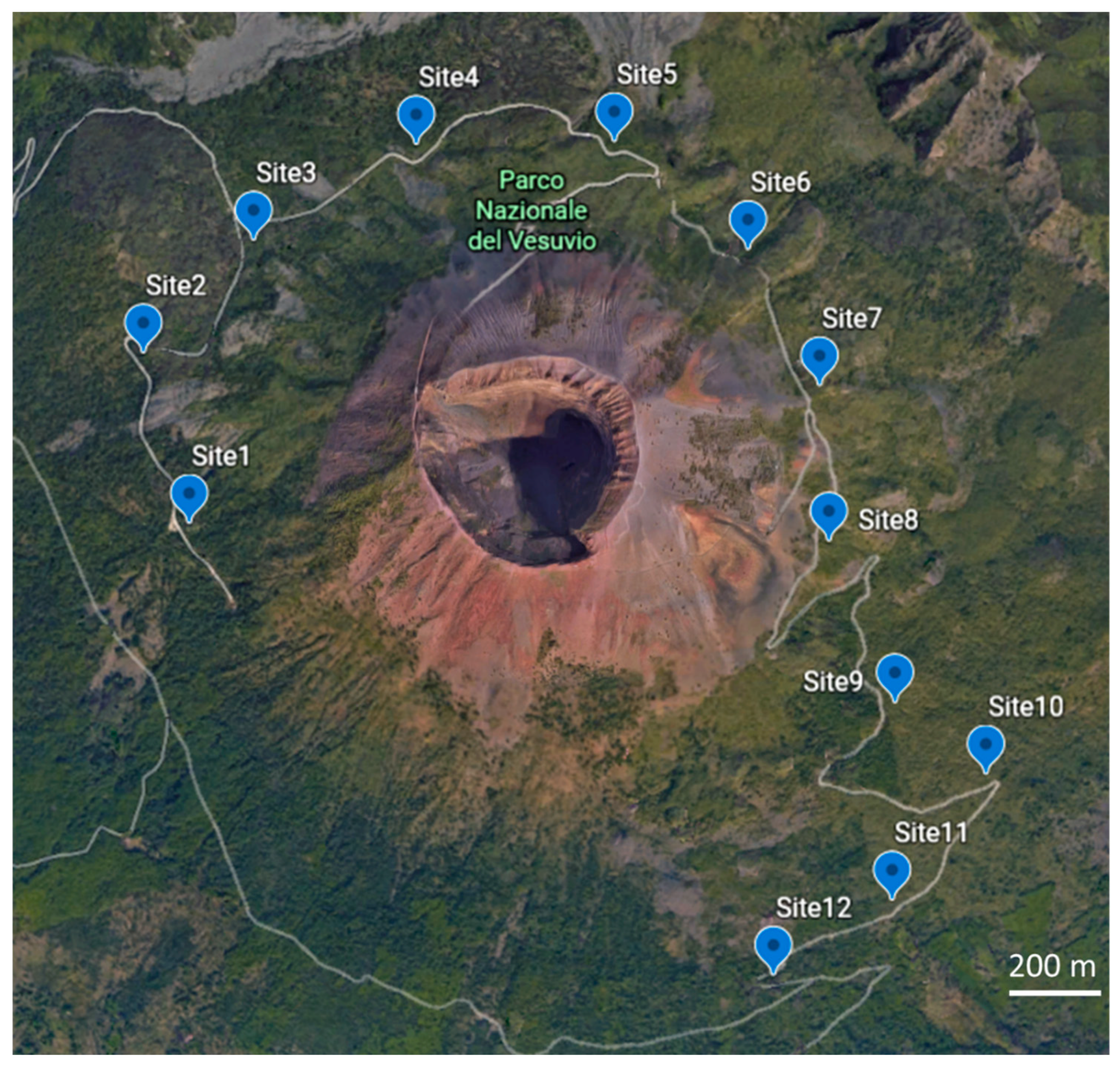This image is a detailed aerial view of Mount Vesuvius, resembling what one might find in a textbook or weather model. The photograph, possibly sourced from a satellite or Google Earth, captures an overhead perspective of the volcano during the daytime. The volcano's central crater, slightly lopsided and approximately an inch in diameter in the image, is surrounded by reddish-brown lower slopes and grayish-brown upper slopes. Encircling the volcano, lush green vegetation interspersed with patches of gray terrain is visible, indicating a rich and diverse landscape. 

Prominently displayed at the top center of the image in green text is "Parco Nazionale del Vesuvio," suggesting that this is an annotated map of the national park surrounding Mount Vesuvius in Italy. Around the crater, starting from the nine o'clock position and circling clockwise, blue balloon-shaped markers designate sites 1 through 12, hinting at various points of interest or trails within the park. In the lower right corner of the image, a white bar indicates a scale of 200 meters, underscoring the vastness of the depicted area. This detailed representation evokes the historical significance of Mount Vesuvius, notorious for the catastrophic eruption that buried Pompeii in 79 AD.